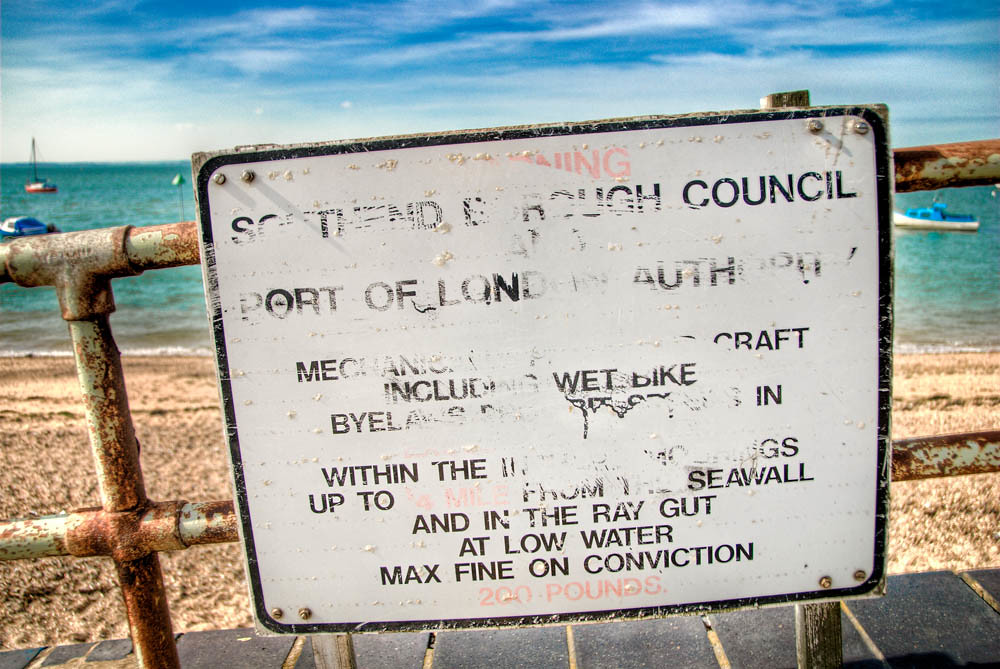The image captures a beachfront scene during daytime with a cloudy sky visible in the distance. In the foreground stands a rusted iron fence that supports an old and weathered white metal signboard, partially covered in black text that's heavily faded and illegible. The signboard features remnants of wording, specifically mentioning "borough council," "Port of London Authority," and "max fine on conviction," with the fine set at 200 pounds. Below the fence, a sandy beach stretches towards a wide, blue ocean dotted with various colored boats; notable among them are a blue and white boat on the right and a red and white boat on the left. The beach and water appear clean and well-maintained despite the rustic state of the fence and sign.